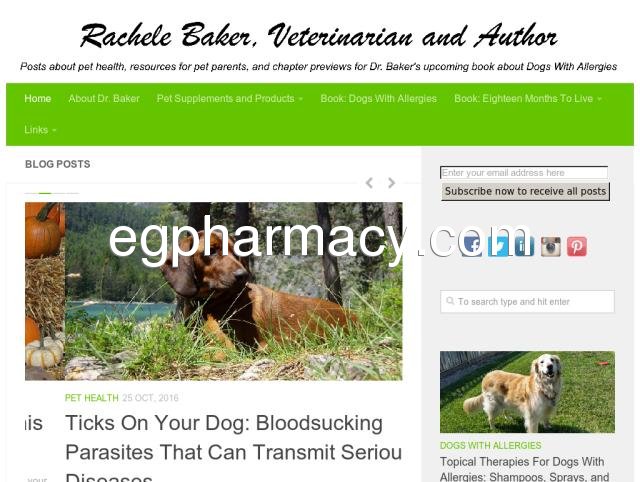Here's a descriptive caption based on the cleaned-up information:

"On a clean white background, at the top center, the text reads 'Rachel Baker, Veterinarian and Author,' followed by a brief description: 'Posts about pet health, resources for pet parents, and chapter previews for Dr. Baker's upcoming book about dogs with allergies.' Below this, a prominent green box contains various links labeled 'About Dr. Baker,' 'Pet Supplements and Products,' 'Book: Dogs with Allergies,' 'Book: 18 Months to Live,' and 'Links,' each accompanied by a small down arrow. Further down, a white box featuring blog posts sits to the side, navigated by left and right arrows.

Dominating the center, there is an image of a large brown dog lying on the ground, surrounded by pumpkins on the left, near a serene little lake with a large tree in the background. Overlaying this image, the text 'echepharmacy.com' appears prominently in white letters. The accompanying caption reads: 'Pet Health, 25th of October, 2016 - Ticks on Your Dog: Blood-sucking Parasites That Can Transmit Serious Disease.'

To the right, a large blue box invites users to 'Enter your address here,' encouraging subscription with the prompt 'Subscribe now to receive all posts.' Below, various social media icons for Facebook, Twitter, and more are displayed. Additionally, there's a search box beneath a picture of another dog standing on grassy terrain, marked by its attractive brown and white fur. The section highlights 'Dogs with Allergies,' detailing 'Topical Therapies for Dogs with Allergies: Shampoo, Sprays, and More.'"